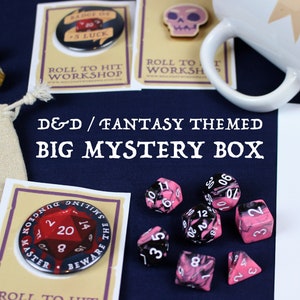The image appears to be an advertisement or cover for a D&D (Dungeons & Dragons) fantasy-themed big mystery box. In the upper right corner, there's a white mug with a brown star emblem. Below the mug are two square-shaped panels, each featuring buttons that read "Roll to Hit Workshop"; one of these panels also has a skull image. Beneath these panels, in white text on a black background, it says "D&D/Fantasy-Themed Big Mystery Box."

In the lower right corner, there are seven dice in various shapes, including pyramids, squares, and octagons, with numbers ranging from 1 to 90. Some of the dice are pink or purple. To the left of the dice, another panel features a button that reads, "Master, beware the smiling dungeon master." This panel also has numbers like 20 on a red background, 2 on a red background, and 14 on a black background. Below that, it again says "Roll to Hit Workshop." The overall background of the image is blue.